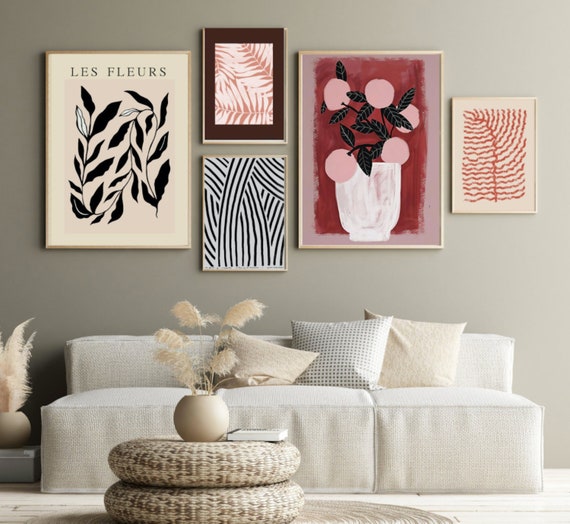The image depicts a sophisticated living room with a beige wall adorned with five art prints. These prints include a black and white piece titled "Le Fleurs," which prominently features two plant stems with dark green and white leaves. Adjacent to it is a stacked pair of prints, the uppermost being a white and peach-colored leaf pattern bordered in red and framed in gold and white, and the lower one has striking blue and white stripes in a gold frame. The fourth print presents a bold portrayal in a pink and red background, showcasing pink spherical objects resembling fruit, black leaves, and a white pot, enclosed in a gold or cream frame. The final print on the far right features orange stripes on a white background with a cream or gold frame.

Beneath the art, a white couch, adorned with three neutral-toned throw pillows, one of which has blue spots, commands attention. In front of the couch is a distinctive coffee table designed like two circles stacked on top of each other, colored in gray and white. The table is accessorized with a book and a white vase containing feathery plants. To the left of the couch, a small block or stool supports another round vase with similar feathery decorations. The room is tied together with a gray rug that lies beneath the coffee table, complementing the overall calm and elegant aesthetic of the space.